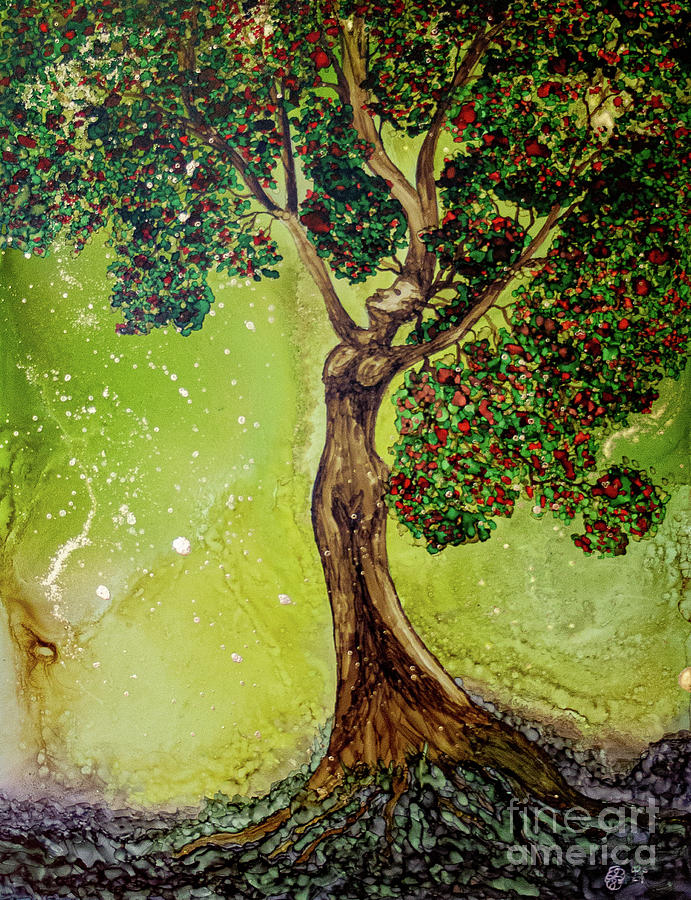The image is an intricate painting of a tree that transforms into a woman, reminiscent of the mythological figure Ariadne. The background is a vibrant blend of bright spring greens and yellows, with white circles scattered throughout, evoking a radiant, lively atmosphere. The ground is a mosaic of teal, purple, and green tones, dotted with what appear to be stones and flowers. The tree's trunk, depicted in various shades of brown, morphs into a female form with her arms upraised, turning into branches. Her hair also extends into the branches, adorned with green leaves and tiny red berries or flowers. The woman's body, seamlessly integrated into the tree’s structure, displays the curves of her form, with her face lighter in color, almost white, giving it a carved, distinct appearance. The painting is signed “Fine Art America” in the bottom right corner in a translucent, gray font.